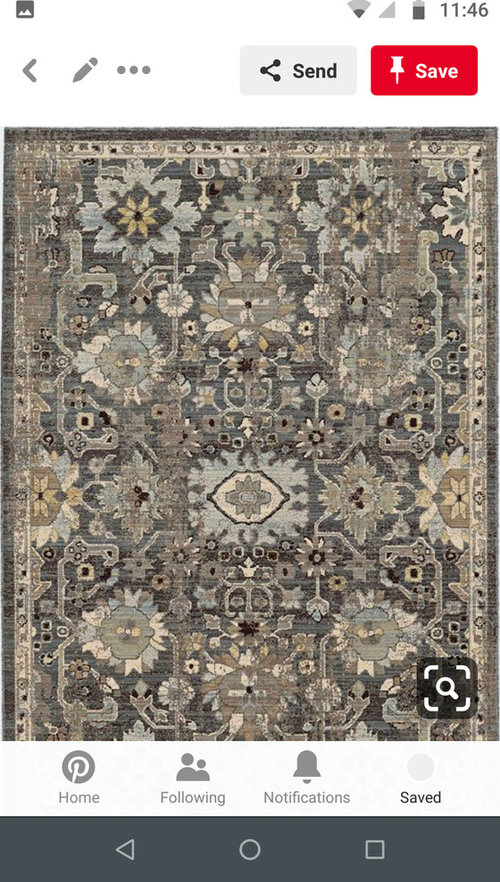The image appears to be a screenshot taken from a mobile phone. In the upper left-hand corner, there is a gray and white picture icon. On the upper right-hand side, various status icons are visible: a Wi-Fi icon that is a quarter full, a signal icon with no bars, and a battery icon at three-quarters capacity. The time displayed is 11:46. 

On the left side of the screen, there is a gray left-pointing arrow, followed by an edit icon, a three-dot menu icon, and a send button labeled "Send." On the right side of this row is a save button with a red background featuring an upside-down thumbtack icon.

Below this, the image shows a section of a rug with artistic designs, resembling a throw rug. The patterned designs are floral-like and feature earth tones, including various shades of brown and stone-like colors.

At the bottom of the image, navigation icons for 'Home,' 'Following,' 'Notification,' and 'Save' are visible.